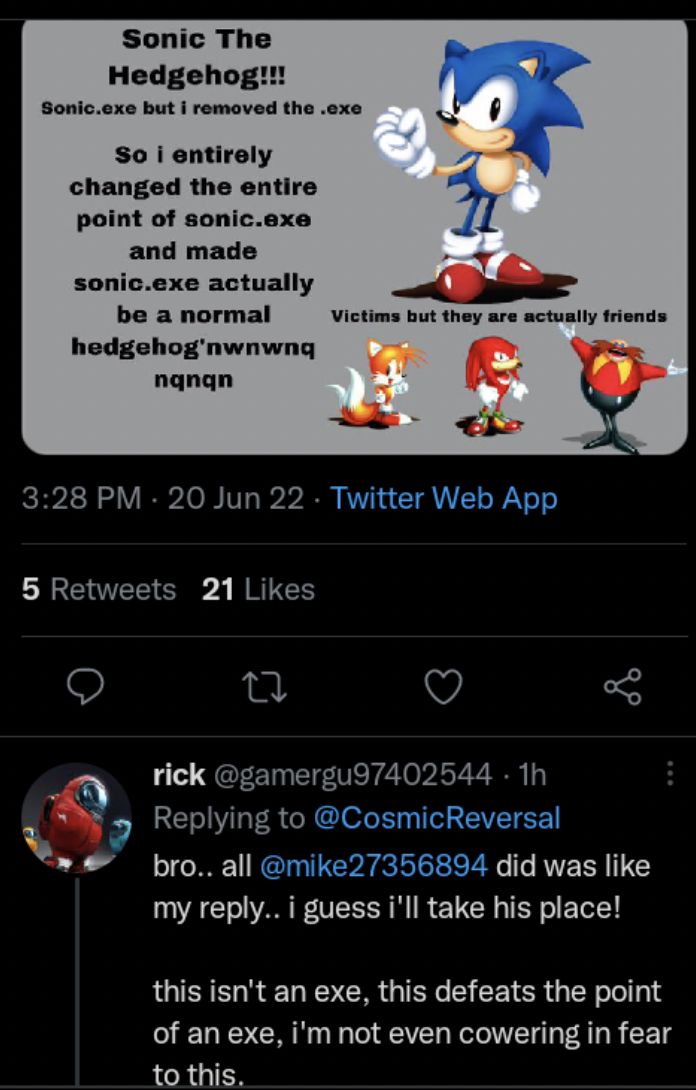This Twitter image captures a lively discussion about Sonic the Hedgehog and a unique twist on the infamous Sonic.exe character. At the top left, "Sonic the Hedgehog" is prominently mentioned. The user discusses removing the ".exe" aspect, transforming Sonic.exe into a normal hedgehog, thereby completely altering the character's sinister narrative. The post itself is characterized by a distinctive stream of text: "NWNWNQNQNQNQNQ."

Below the text is an image of Sonic the Hedgehog—a lively blue hedgehog wearing red shoes and white gloves. The caption under the image amusingly refers to "victims," though they are actually Sonic’s friends: Tails, a two-tailed fox, and Knuckles, a red echidna with white gloves and shoes. The notorious villain, Dr. Eggman, is also featured, described as egg-shaped with a bald head and a red mustache.

Further details of the tweet indicate that it was posted at 3:28 p.m. on June 22 via Twitter's web app, garnering 5 retweets and 21 likes. The interactions include a reply from Rick (@GamerGU974025441), commenting about the pointlessness of removing the `.exe` element, stating, "This isn’t an exe; this defeats the point of an exe. I’m not even cowering in fear to this." The reply was directed towards @cosmicreversal and @Mike27356894.